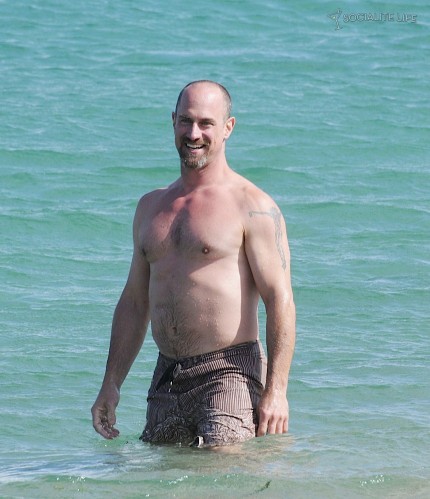In this image, we see a bald man standing in the ocean, his legs submerged up to his thighs in the turquoise, clear, calm water, with only minor ripples surrounding him. He has a small goatee with a mix of gray and brown hairs and a slightly rounded, fair-skinned belly. His hair is short on the sides, and he is shirtless, which reveals a tattoo on his upper left arm. The tattoo resembles a person with arms outstretched, possibly depicting a crucifix. He is wearing beige brown swim trunks that reach his thighs, and there's a hint of sunburn on his chest and neck. The day appears sunny, as the bright sunlight is evident on his skin and the water surface. He is smiling warmly at the camera.